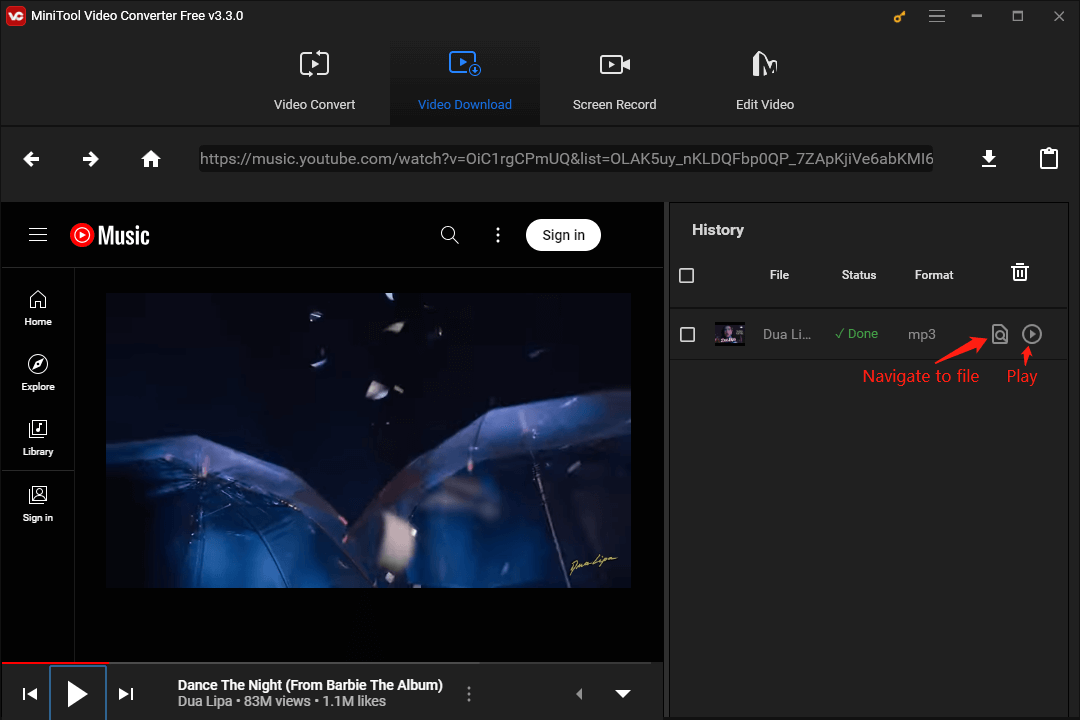This image appears to be a screenshot from YouTube Music, characterized by its black background interface. At the top, several options are displayed: "Video Convert," "Video Download" (which is currently selected, indicated by a black box and blue highlight), "Screen Record," and "Edit Video." The screen shows the music video for "Dance the Night" by Dua Lipa from the Barbie album, boasting 83 million views and 1.1 million likes. The viewer is not signed in, as evidenced by the presence of a "Sign In" button. Below the video, a history panel lists the song file. The status reads "Done," the format is MP3, and red text with an arrow points to the "Navigate to File" and "Play" options, suggesting a tutorial or guide. Additionally, navigation buttons such as "Back," "Forward," and "Home," along with the URL of the current page, are visible at the top of the screen.